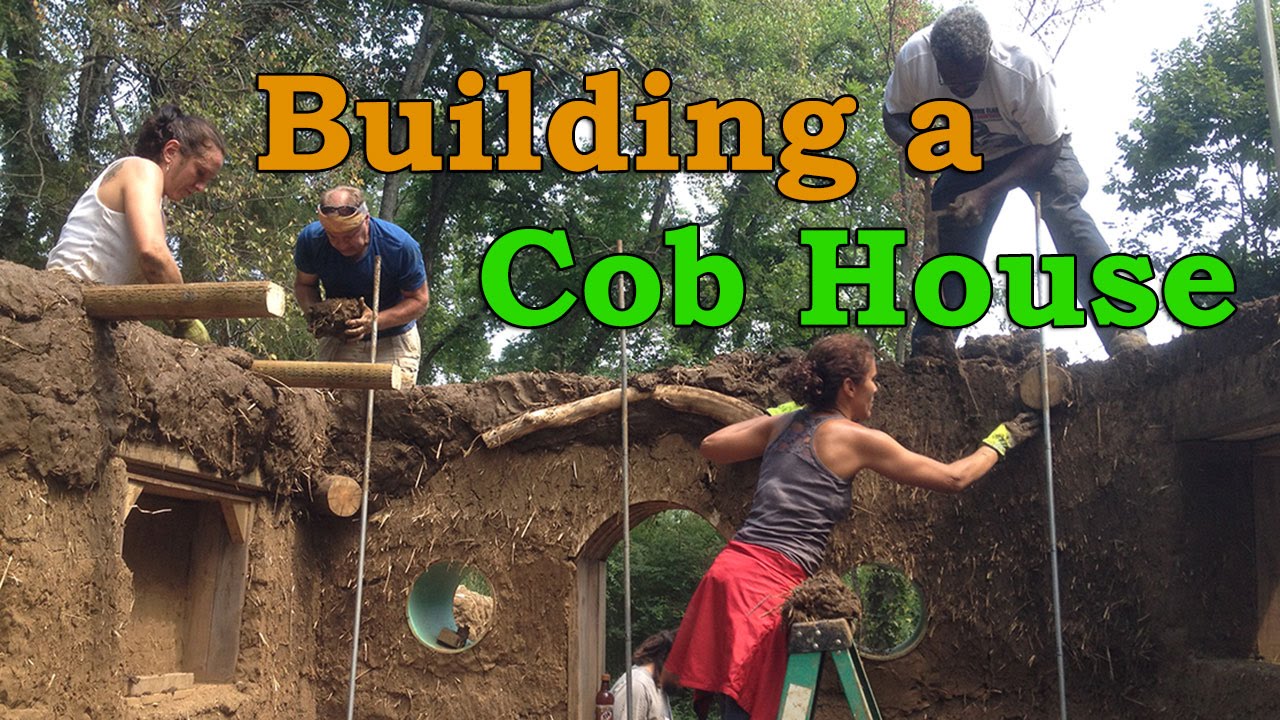The image is a still frame from a video or a banner, showcasing people constructing a cob house. The scene depicts four individuals actively working on the structure, which resembles a roofless mud hut with an array of circular windows and a door framed in wood. The house occupies the bottom half of the image, displaying three significant poles for support and a woman positioned on a ladder in the middle, contributing to the top of the wall.

In the top half, a black man stands on the right, holding a device likely used for tamping down the wall. To the left, an older bald man works alongside another woman, both focusing on the wall's construction. The background consists of trees with patches of sky visible, enhancing the outdoor setting's rustic ambiance.

Large, classy text across the top reads "Building a Cob House," with "Building A" illustrated in orange with a black outline and "Cob House" in lime green with a black outline. The detailed setting, materials, and vibrant text suggest this could be a YouTube video thumbnail, reflecting both the community effort and the earthy, sustainable building process.

The cob house appears to be constructed with mud and straw, highlighted by supportive wooden beams and detailed work around window frames and doorways. The scene exudes a sense of teamwork and enjoyment among the builders.